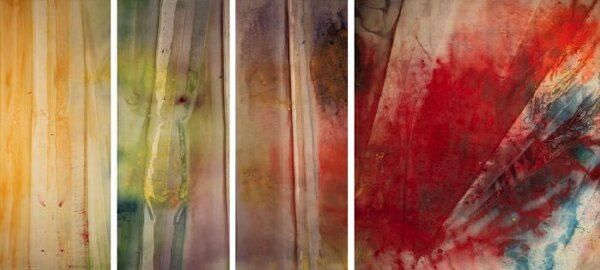The image is an abstract painting composed of four distinct sections, each resembling lengths of wood, which could invoke the idea of a fence. The leftmost three sections are vertical rectangles of identical size, approximately 2-by-4 units, while the rightmost section is a nearly perfect square, double the width of the others but just as tall. 

The first section on the left features streaks of light and dark yellow, with occasional flecks of red and green, painted in an organic, non-rigid manner. 

The second section displays the natural grain of the wood subtly leaning to the right, with blotchy, uneven patches of vivid green paint and hints of yellow. This section also contains traces of lighter red and a gradient that fades into purple.

The third section exhibits purple and red splotches, along with some black accents, over a background that includes pinkish hues and bits of tan.

Finally, the larger square section on the right is dominated by a central splash of bright red paint, which disperses outward in a dynamic splatter pattern. There are also significant areas of light blue underneath the red, particularly noticeable on the right side, and a single unpainted spot near the top that reveals the dirty white background of the piece.